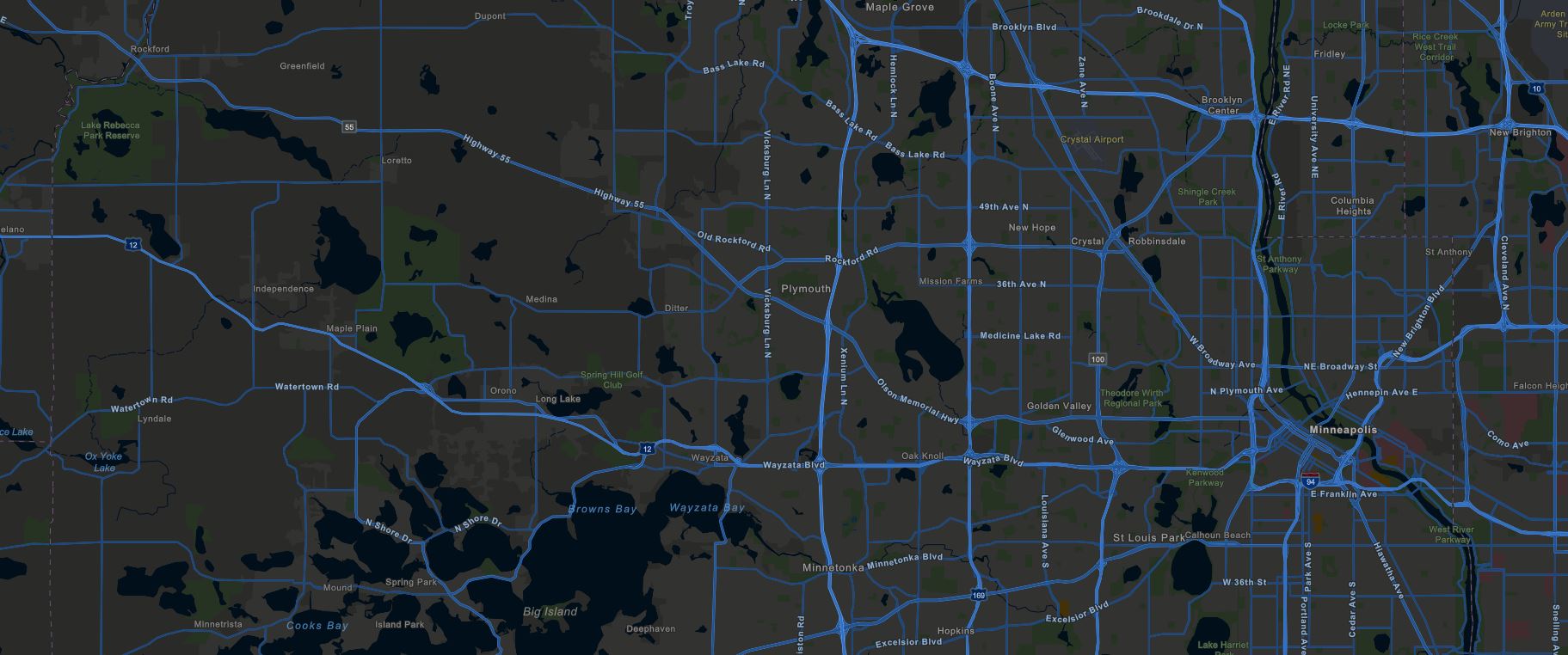The image is a rectangular map of Minneapolis, oriented from left to right, with a balanced proportion—not super thin, yet not overly large. The background is composed of various shades of gray, ranging from lighter tones to darker, almost black patches, which signify bodies of water scattered throughout the map. Interspersed throughout the gray background are patches of green, indicating parks or natural areas.

Prominently featured across the map are numerous blue lines, which are curvy and meandering, representing the city's waterways. These lines are not straight but rather filled with dips and waves, adding to the dynamic flow of the map's layout.

Along these blue lines are the names of different towns and neighborhoods, marked in white letters. Notably, Minneapolis is labeled towards the right side of the map. In addition, some place names are highlighted in a yellowish color, differentiating them from the rest.

Overall, the map intricately combines color and text to depict the geographical and urban layout of Minneapolis, with its water bodies, green areas, and detailed labeling of various locales.